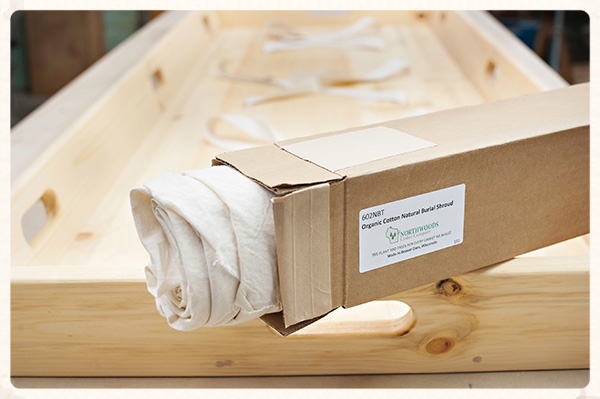The color photograph captures a detailed scene involving multiple elements arranged with care. At the center, a long brown cardboard box labeled "602 NBT Organic Cotton Natural Burial Shroud, Northwoods" is prominently displayed. The box, tilted towards the left, is open at one end, allowing a rolled piece of burlap-type fabric to partially emerge. This cardboard box rests on a light-colored wooden tray that features handles and natural tie straps adorning its base. The wooden tray itself sits atop another wooden table, creating a layered effect. The image focuses entirely on these objects, with no people present, highlighting the juxtaposition of the natural materials and the orderly arrangement.